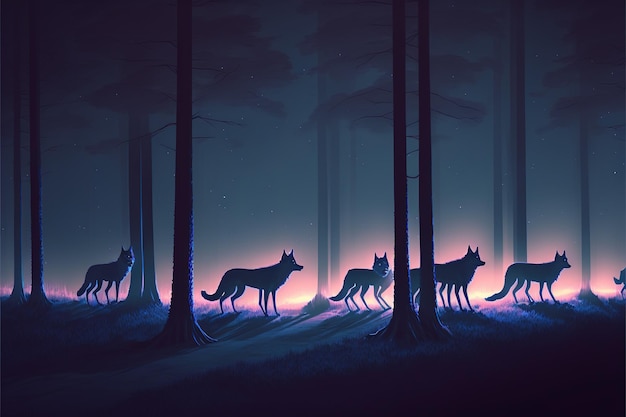This is a digitally created nighttime painting set in a deciduous forest. The scene features a dark, blue sky speckled with a few white stars and dark clouds. Twelve tall, bare trees with brown branches stretch across the landscape, adding to the eerie ambiance. In the foreground, there are six wolves standing in a group, their profiles silhouetted against an intense orange and yellow light that floods the horizon. This light, possibly emanating from a fire, casts a haunting glow throughout the picture. There is also a hint of purple near the bottom of the composition, adding depth to the scene. Despite the serene beauty of the artwork, the implications of a forest fire approaching the wolves add a layer of tension and urgency to the image.